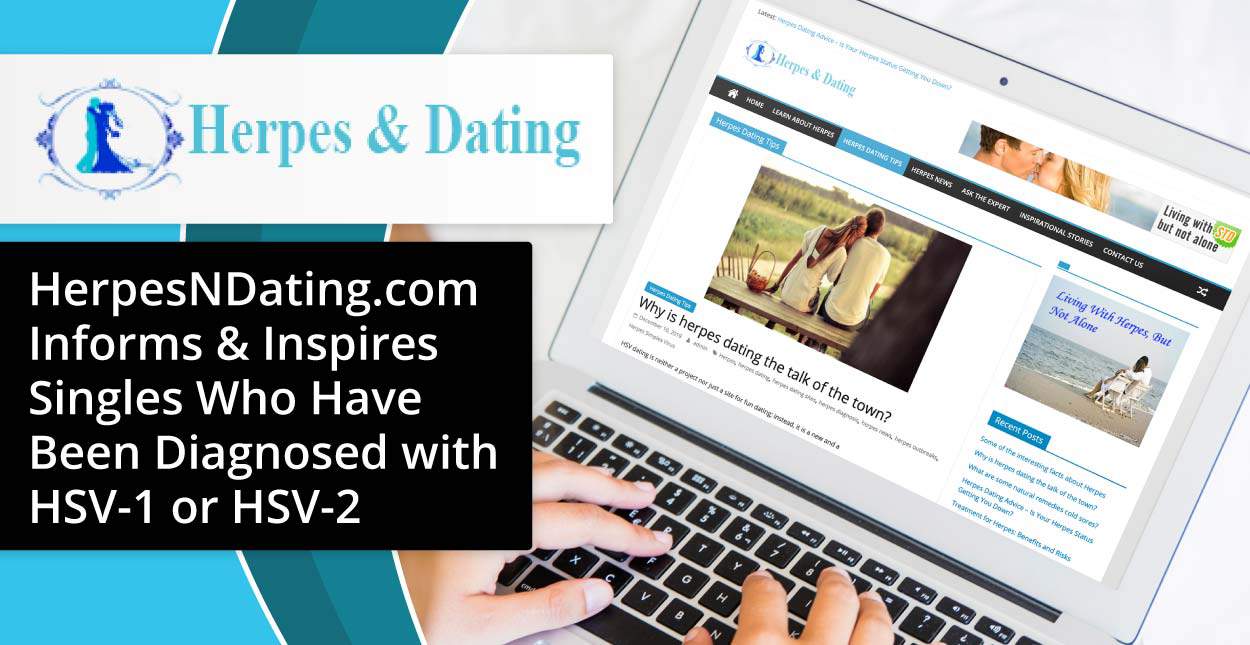The image depicts a laptop open to the "Herpes and Dating" website. Only the hands of the person typing on the keyboard are visible. To the left of the image is a white rectangular box with the text "Herpes and Dating" in aqua blue font, accompanied by a logo on its left. Below this, a black box with white font provides a tagline: "herpesanddating.com informs and inspires singles who have been diagnosed with HSV-1 or HSV-2." The predominant background behind the laptop is a whitish-gray, while a circular area in a greenish-blue hue appears to the left. The far left of the site features an aqua blue gradient, adding a colorful contrast to the overall image.